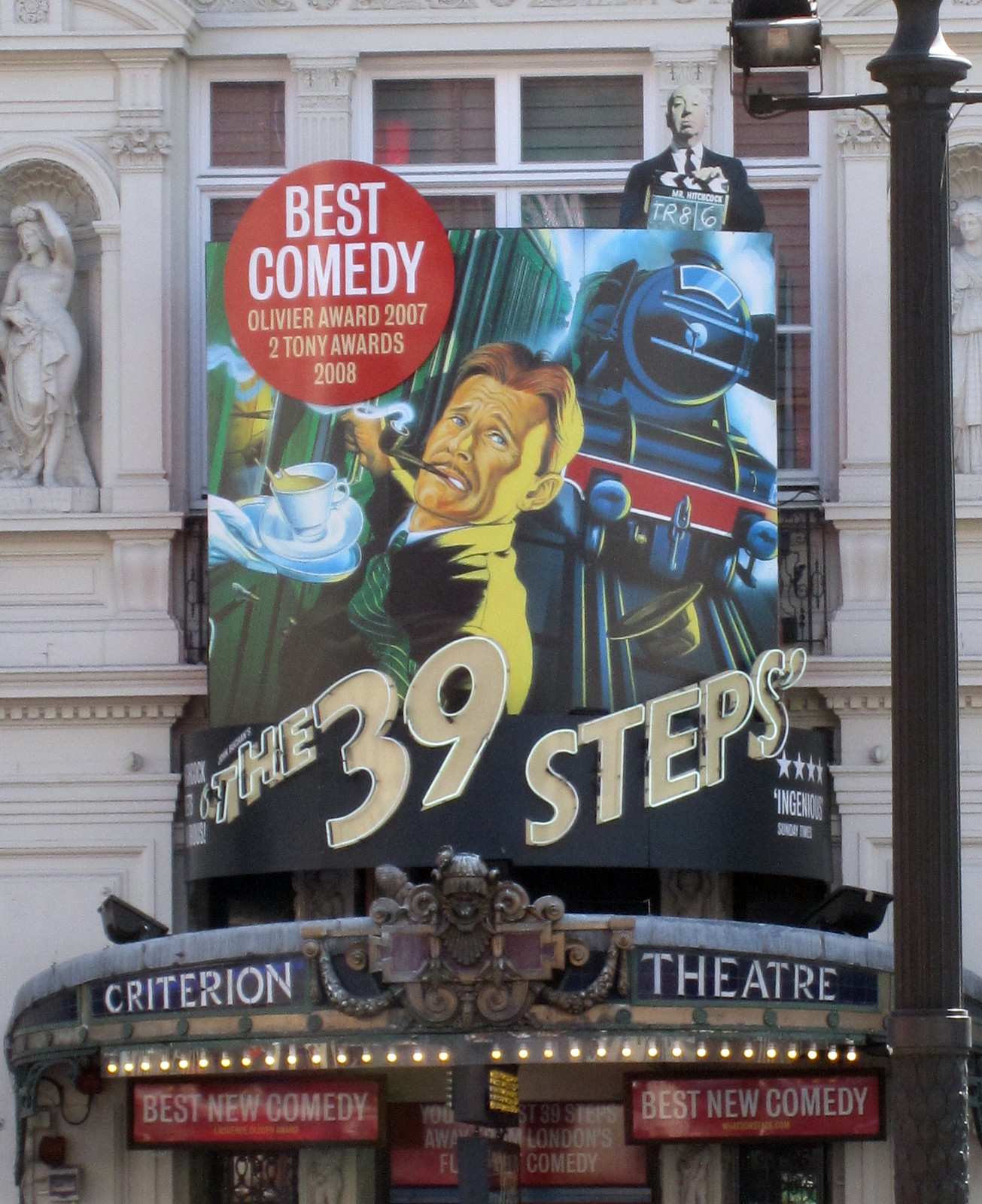In this tall, rectangular image of a movie theater entrance, a grand off-white building with a statue of a woman in a large fabric dress, standing under two columns, anchors the background. Below, the old-fashioned, intricately designed awning displays the theater’s name in white tiles on a black background: "Criterion Theater." Above this, another awning, black with beige letters rimmed in lighting, announces "The 39 Steps," accompanied by an image of a man smoking a cigar on a train. An elaborate poster above highlights "Best Comedy" in white on a red circle, referencing the "Oliver Award 2007" and "Tony Awards 2008," featuring the same man with a cigar, holding a coffee cup, as a train approaches. The upper right corner of the poster depicts Alfred Hitchcock's image. Below the Criterion Theater marquee, two red signs on either side also declare "Best New Comedy," contributing to the inviting, historical feel of the theater's presentation.